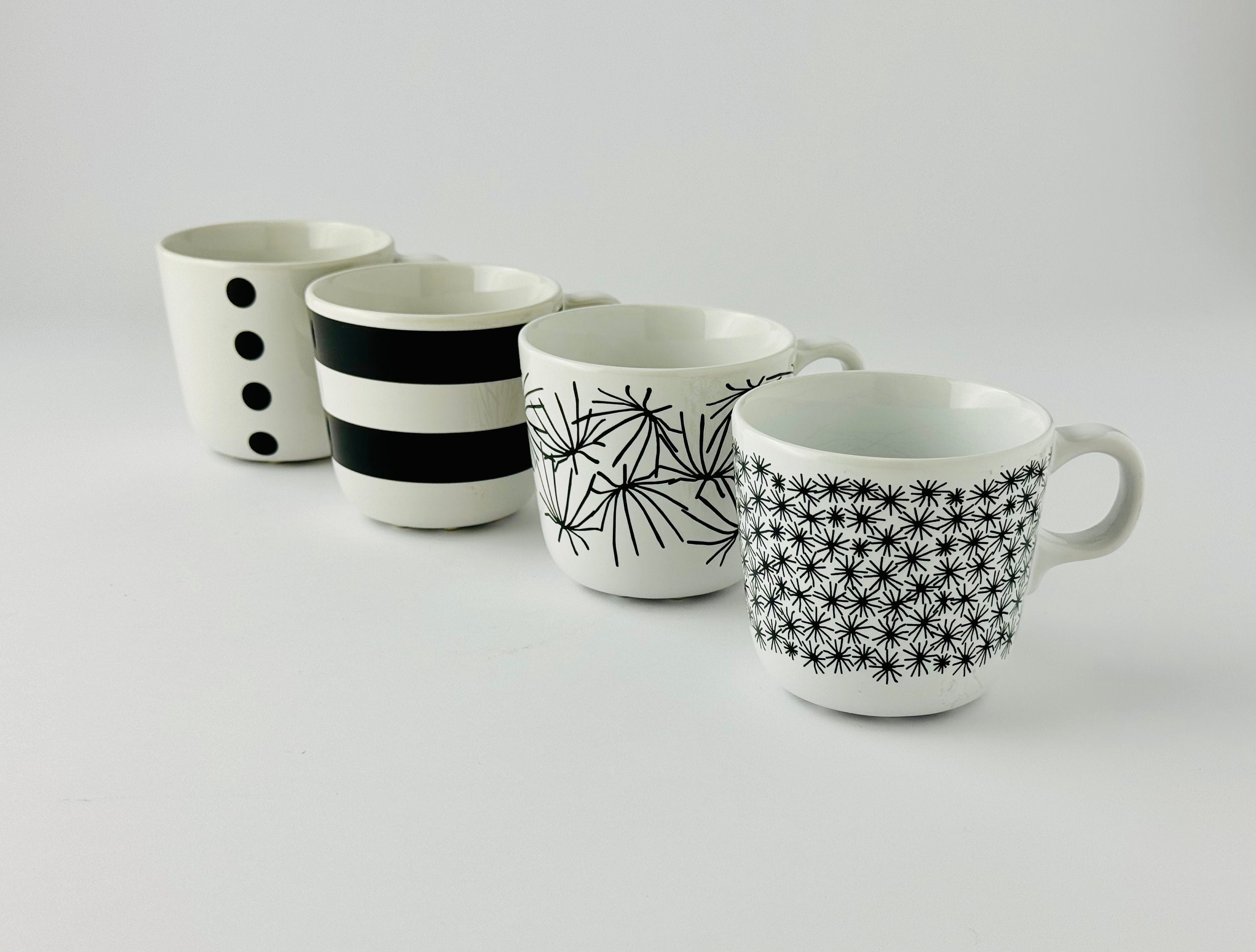This detailed photograph showcases a collection of four coffee mugs, meticulously arranged diagonally from the top left to the bottom right corner against a light gray background. Each mug is uniform in size, featuring distinctive designs on their white handles and body. 

Starting from the top left corner, the first mug is pure white adorned with a vertical arrangement of four black polka dots. Moving to the second mug, bold and thick black and white horizontal stripes wrap around its surface, creating a striking visual contrast. The third mug in the lineup presents a more delicate aesthetic, its design resembling floral patterns or blades of grass, although upon closer inspection, these elements recall elongated black shapes akin to spider legs, each surrounding a shaded black center. Lastly, the mug positioned at the bottom right is covered in an intricate, denser floral pattern, evoking an astral or celestial motif. 

The handles of all mugs are white and oriented to the right, and the insides of these mugs are empty, highlighting their pristine presentation. The entire set, devoid of any border or text, emphasizes the beauty and diversity of the crockery designs.